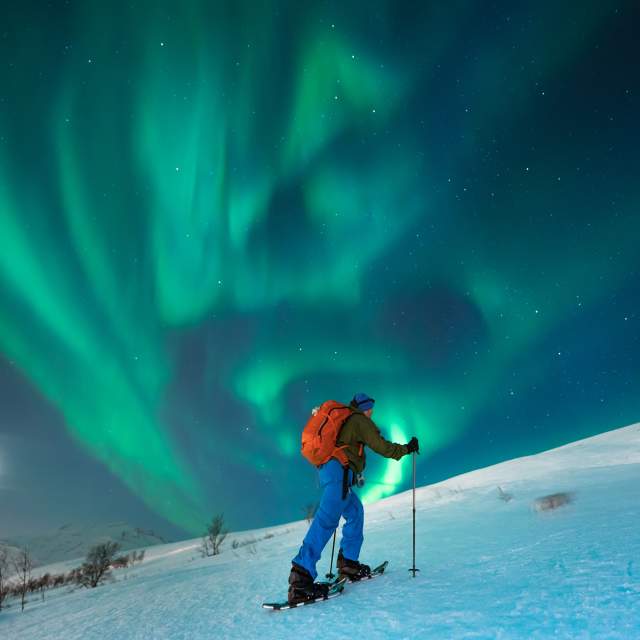A photograph captures a person trekking uphill in the snow, equipped with snowshoes designed to prevent sinking into the white, powdery snow. They are using walking sticks that resemble ski poles for assistance. The climber is dressed in royal blue pants and a brown long-sleeved shirt, topped with a blue knitted cap. Black gloves protect their hands, and a large, bright orange backpack rests on their back. The striking sky above features a rich mint green light reminiscent of the aurora borealis, interspersed with white speckles of stars. A bold blue and black starry expanse serves as the backdrop to this otherworldly glow. Scrawny bushes dot the background of the snowy landscape, adding to the serene yet surreal quality of the scene.